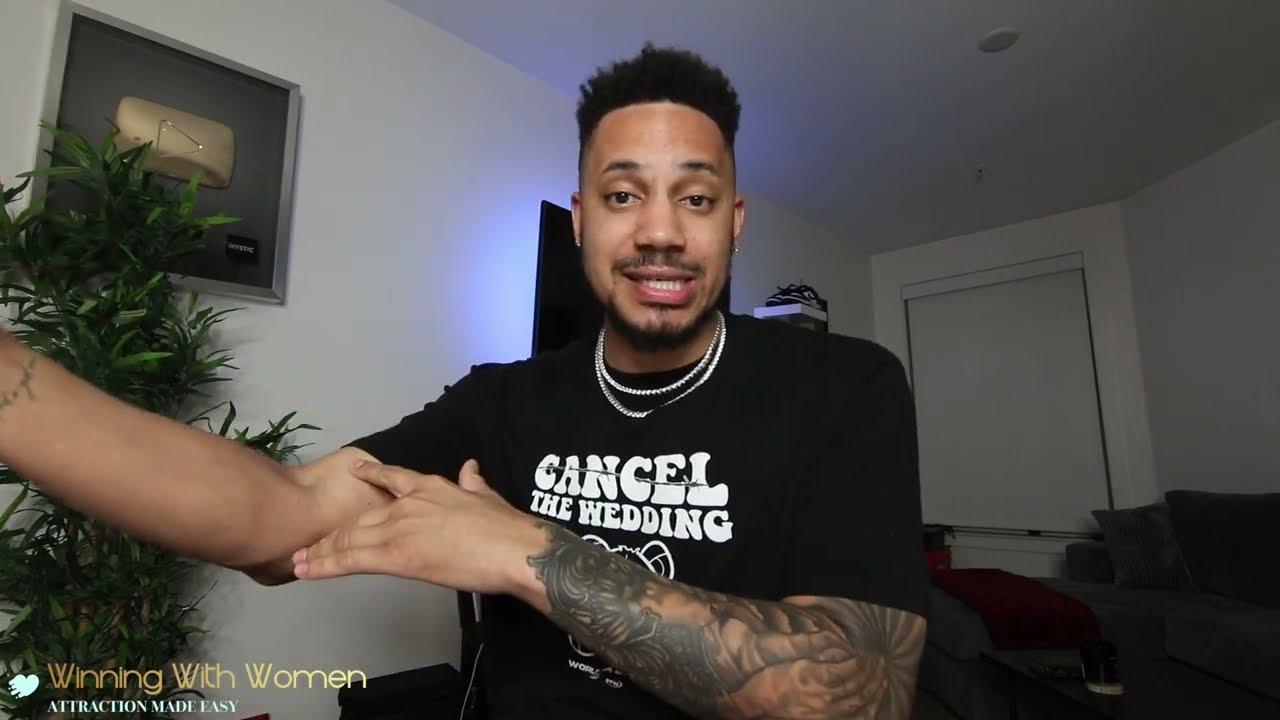The image captures a black man with a tall, shaved hairstyle, known as a Gumby haircut, standing in a well-lit room with white walls and white blinds covering the windows. The room's ceiling features a fire sprinkler and a light fixture. The man sports a black t-shirt that says "Cancel the Wedding" and is adorned with two necklaces. He has a large tattoo that extends down his left arm, stopping at the wrist, which also bears a smaller tattoo with indiscernible writing. His right arm is raised, pointing at his left arm, and he wears an earring.

The man appears to be talking, with a peculiar smile and open mouth, seemingly looking slightly downward at the viewer. Behind him, a red couch with pillows is visible, along with a sizable potted plant to his left. The wall behind him displays two frames: one black and the other containing something white. A black sofa and a doorway can also be seen in the background. Additionally, a YouTube award is mounted on the left-hand side wall above the plant. A blue light suggests the scene might be shot at night. In the lower left corner of the image, the text "Winning with Women - Attraction Made Easy" is displayed.